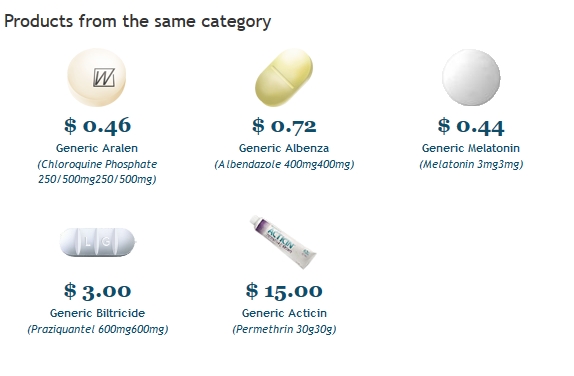The image appears to be a screenshot from a pharmaceutical website listing various medications against a white background. At the top of the image, there are products from the same category. Below, the list of different medications is displayed with the following details:

1. Top left: A white, circular pill imprinted with a "W." The price is $0.46 and it is labeled as generic Aralen, available in 250-500 mg doses.
2. Next: An oval-shaped, beige-colored capsule priced at $0.72, described as generic Albenza.
3. Following that: Another white, circular pill priced at $0.44, labeled as generic Melatonin.
4. Below: An oval-shaped pill with lines on it, priced at $3, and identified as generic Biltricide.
5. Final: A tube priced at $15, labeled as generic Acticin.

This detailed description ensures clarity and specificity for each medication listed in the image.